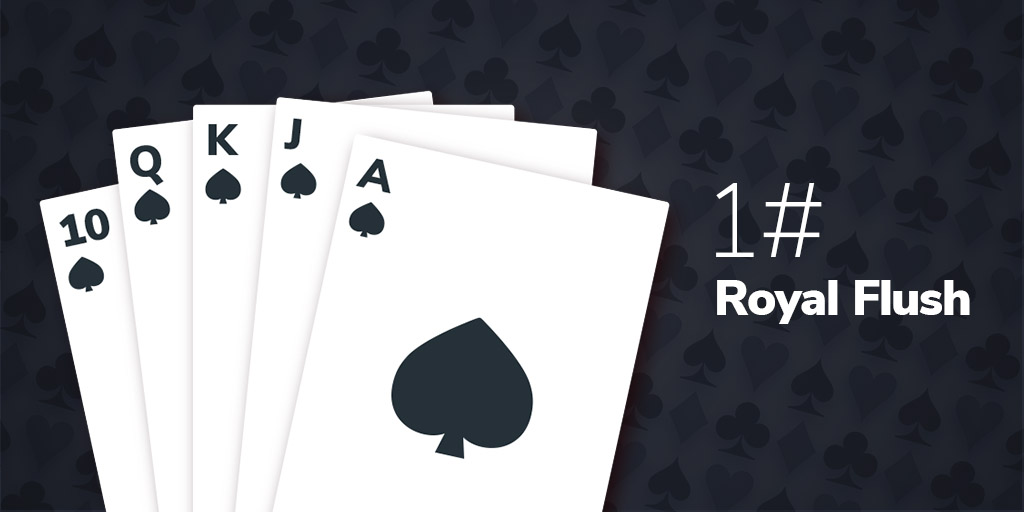The image features five playing cards, each white with black graphics, arranged in an overlapping row from left to right: the 10 of spades, queen of spades, king of spades, jack of spades, and ace of spades. The background is a navy blue color with a repeating pattern of card emblems. To the right of the cards, white text reads "£1" in a light, thin font, followed by "ROYAL FLUSH" in bold, white text. The overall design suggests an advertisement, prominently highlighting the theme of a card game with a royal flush hand.